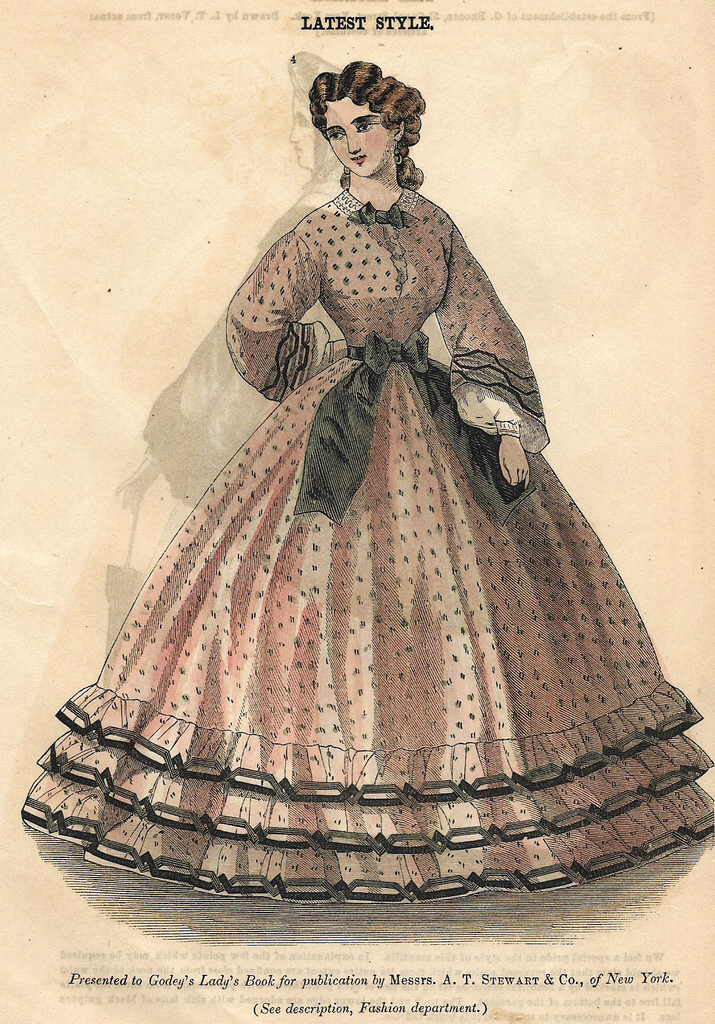This detailed illustration, set against a beige parchment-style background, features the words "Latest Style" prominently at the top, indicative of its antique origin, likely a late 19th or early 20th-century publication. It is presented to Godey's Lady's Book for publication by Monsieur A. T. Stewart & Company of New York. The focal point is a drawing of a woman in an elaborate, flared, three-tiered ball gown, predominantly pink with black or dark gray polka dots. The dress is cinched at the waist with a thick black sash and adorned with three buttons down the chest, accentuated by a bow tie. The voluminous sleeves, edged with intricate black lace, billow out gracefully. The hem of the gown also features black lace ruffles. Additional intricate patterns interweave black and gray around the cuffs of the sleeves. The woman's long brownish-red hair is styled with a slight head tilt to the left, accompanied by a gentle smile on her face. Lingering ink from an adjacent page subtly ghosts through the parchment, adding to the vintage feel of the advertisement.